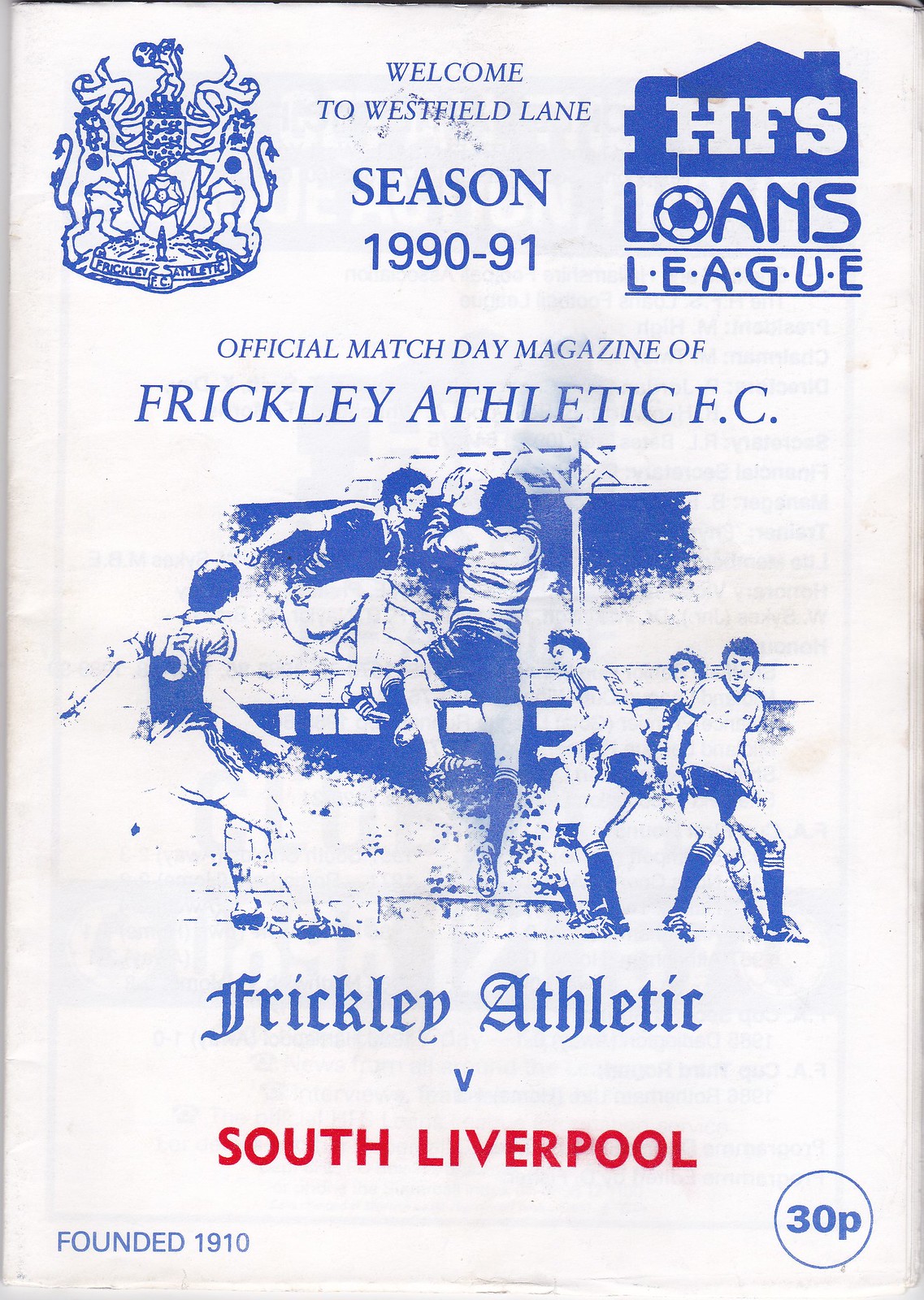The image is of an aged, off-white poster or program with blue text and illustrations. It features a decorative coat of arms in the upper left corner, depicting two lions standing on their hind legs facing each other with a stand between them. On the top right, there is a logo that includes a house symbol with the letters "HFS" in white, followed by the text "Loans League," where the "O" in "Loans" is represented by a soccer ball.

At the center of the poster, the text reads "Welcome to Westfield Lane" in small blue letters, and beneath it, "Season 1990-91" in darker blue. Directly below, it proclaims, "Official Match Day Magazine of Frickley Athletic FC" in larger blue letters.

The lower part of the poster includes a detailed artist's rendering of a soccer match, drawn in blue ink, showing a group of boys playing soccer. This illustration is centered on the page. Beneath this image, the poster text indicates the match between "Frickley Athletic v. South Liverpool," with "Frickley Athletic" and "South Liverpool" in blue text, separated by a red "v."

In the bottom left corner, the poster notes "Founded 1910," and in the bottom right corner, the price is listed as "30 pence."